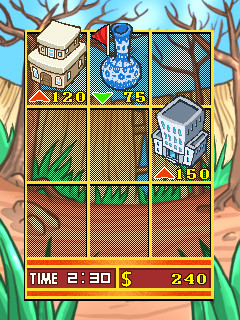This image depicts a video game interface, featuring a 3x3 grid with a yellow outline. Each cell of the grid is filled with a semi-transparent gray color. Three cells contain objects accompanied by numerical values and directional arrows:

1. **Top Left Square**: A two-story building is displayed with a red upward arrow beneath it, alongside the number "120".
   
2. **Top Middle Square**: A blue and white vase with a red flag is shown, accompanied by a green downward arrow and the number "75".
   
3. **Middle Right Square**: A skyscraper is illustrated with a red upward arrow, along with the number "150".

Below the grid, the game interface indicates the current time as "2:30" and displays a currency amount of "$240". The background features a scenic landscape with trees, grass, a fence, and a blue sky filled with clouds.